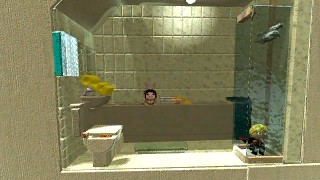In a video game setting, the scene captures a detailed bathroom space. On the left side of the image, there's a speckled wall that contrasts with a backdrop of tiled surfaces. Positioned centrally in the scene, a person is sitting in a brown bathtub. At the bottom left, there is a woven basket acting as a wastebasket. Above this, a white and green towel hangs over a pole, adding another splash of color.

The lighting in the image creates an atmospheric depth, with pronounced darkness at the top and bottom of the scene, while a bright light illuminates the tiled wall in the background. On the far right, there appears to be a glass-enclosed shower or possibly an aquarium, as small fish are visible floating at the top. A person with yellow hair, fair skin, and dressed in black clothing stands at the bottom of this enclosure. Next to the bathtub is a figure referred to as a "bath man," complementing the eclectic mix of elements that make up this quirky, immersive bathroom scene.